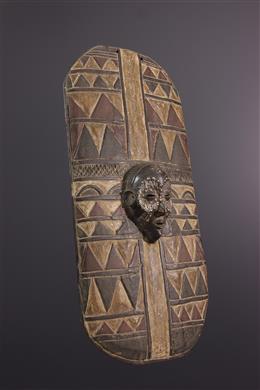This photo features an old, intricately designed African tribal shield made entirely out of wood. The shield is large, approximately the size of a person's torso, and adopts a pill-shaped form with rounded top and bottom ends. Its surface showcases a striking pattern of geometric triangular designs in contrasting shades of dark brown and black, overlaying a lighter wooden background. The centerpiece of the shield is a detailed wood carving of a face, reminiscent of a mask, with distinct features such as eyes encircled by carved divots, ears, and a bald head. This carved face, solid black in color, exudes a fierce expression. The entire artifact rests against a black background, highlighting its aged yet meticulously crafted appearance.